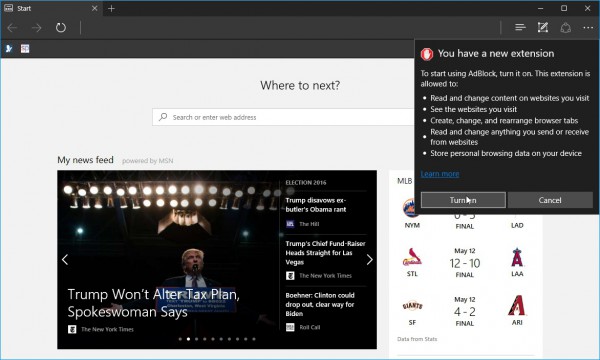The image depicts a search page interface, likely within a web browser, although the specific browser or website is not identifiable from the image. The page is encased in a border, featuring a black banner at the top that includes a start button, directional arrows, a circle icon, an X, and a plus sign.

To the right, there is a prominent pop-up notification resembling a stop sign with a white hand symbol. The notification states: "You have a new extension. To start using Adblock, turn it on." Below this message is a list of permissions the extension requires, along with options to "Turn On" or "Cancel."

The main body of the page has a light blue background. In dark text, it reads, "Where to next?" accompanied by a prominent white search bar. Below this, the text "My News Feed powered by MSN" appears.

Within the news feed section, various headlines and images are displayed. One notable image features Donald Trump, alongside the headline: "Trump won't alter tax plans, spokeswoman says," attributed to The New York Times with its iconic logo. To the right of this image, there are three additional headlines:

1. "Trump disowns ex-Butler's Obama rant" - The Hill
2. "Trump's chief fundraiser heads straight for Las Vegas" - The New York Times
3. "Boehner: Clinton could drop out, clear way for Biden" - Roll Call

Adjacent to these articles are some graphics showcasing icons for different sports teams, including the New York Mets, Arizona, and St. Louis, along with their corresponding sports scores.